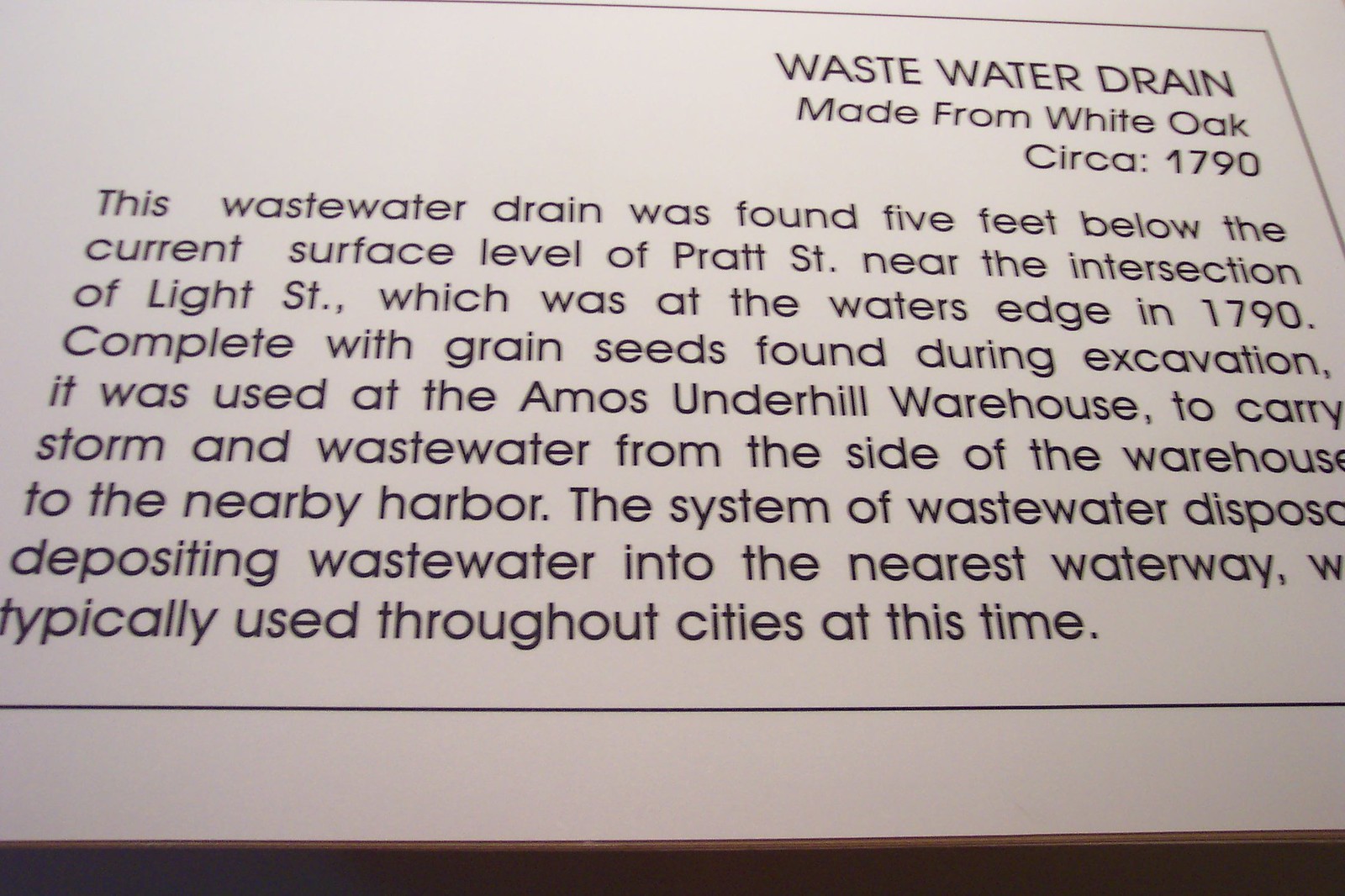This image features a close-up of a piece of paper or board displaying a detailed paragraph about a historical wastewater drain. In the top right corner, the text, in bold all-caps, reads "WASTEWATER DRAIN". Below it, in smaller caps, it states "MADE FROM WHITE OAK, CIRCA 1790". The main body of the text, starting on the left side, informs the reader that this wastewater drain was discovered five feet below the current surface level of Pratt Street, near the intersection of Light Street, which, in 1790, was at the water's edge. During the excavation, grain seeds were found, indicating the context of its use. This drain was a key part of the Amos Underhill Warehouse infrastructure, facilitating the transportation of storm and wastewater from the side of the warehouse to the nearby harbor. This method of disposing wastewater by depositing it into the nearest waterway was commonly used in cities during that period. The paragraph is slightly cut off at the end, leaving the final word incomplete.